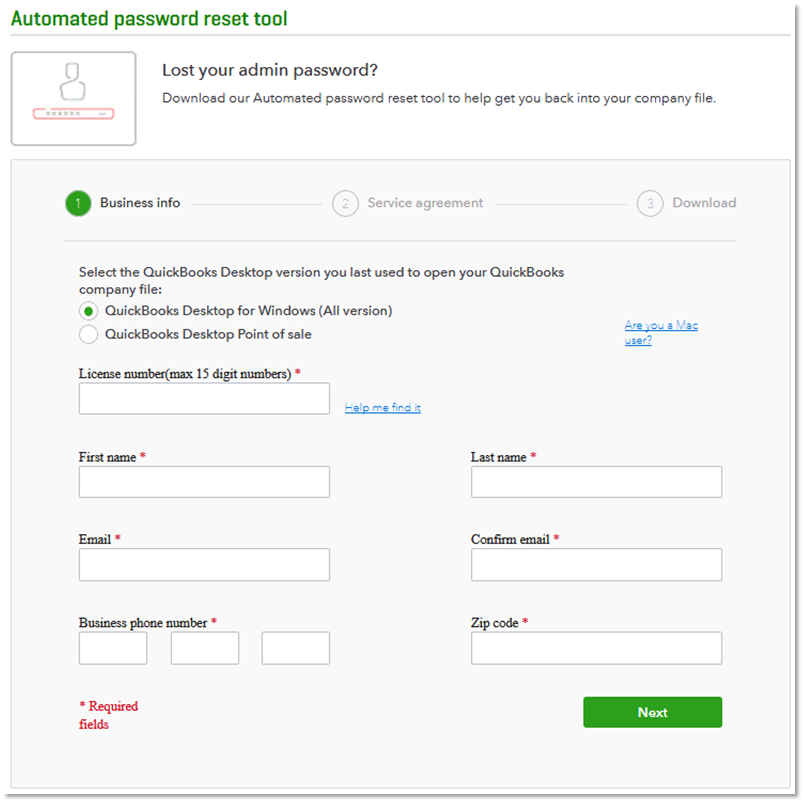### Detailed Descriptive Caption:

This is a screenshot of a webpage dedicated to providing an automated password reset tool for QuickBooks users who have lost their admin passwords. At the top of the page, there is a navigation menu with highlighted 'Business Info' and 'Service Agreement Download' options. The primary content guides users through the process of selecting the appropriate QuickBooks Desktop version they last used to open their company file, specifying that it is for 'QuickBooks Desktop for Windows - All Versions,' excluding Point of Sale.

The form in focus requires users to enter several pieces of information: 
- License Number (with a prompt: 'Help me find it')
- First Name (required)
- Last Name (required)
- Email Address (required)
- Confirming Email Address (required)
- Business Phone Number (required)
- Zip Code (required)

These fields are mandatory to proceed with recovering the lost administration password. The page aims to assist users in regaining access to their QuickBooks company file, emphasizing the importance of having accurate information to successfully reset the password and continue using QuickBooks software.